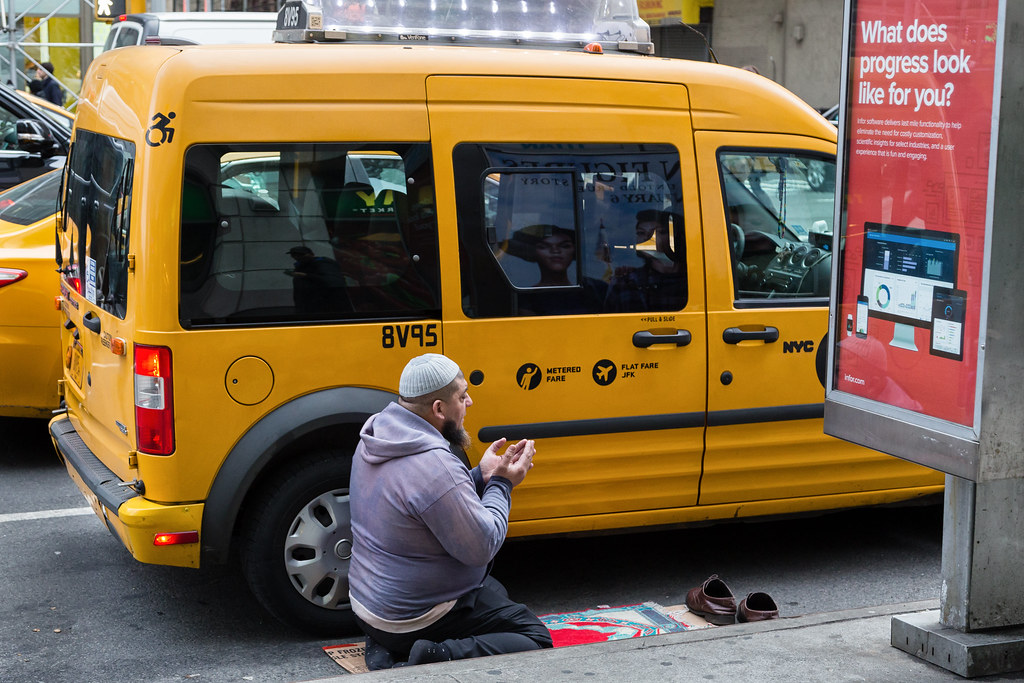The photograph shows a man kneeling on the road near the edge of what appears to be a busy street in Manhattan, possibly during a stoplight. He is engaged in prayer, kneeling on a prayer rug with his palms facing up as if in supplication. The man is wearing a white skull cap, a light blue hoodie, dark pants, and dark socks. In front of him are his brown leather shoes, which he has removed for the prayer. To his left are two yellow taxi vans, one bearing the identification number 8V95. The taxis' design suggests they are accessible vehicles, often used in metropolitan areas like New York City. To his right is a sidewalk, and just beyond that, an electric banner in red reads, "What does progress look like for you?" The overall setting is clearly urban, highlighting the convergence of daily life and personal devotion amidst the hustle and bustle of the city.